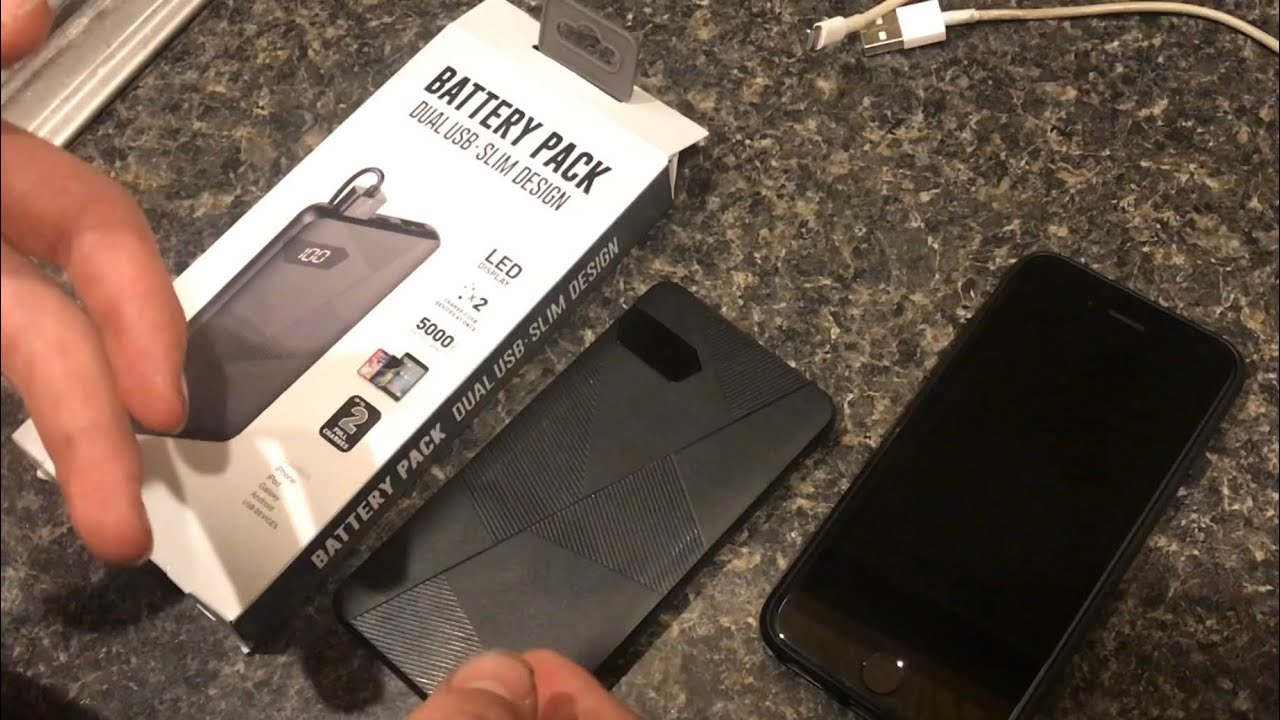In the image, a pair of hands are opening a white box with black bold text that reads "Battery Pack, Dual USB, Slim Design." The left hand is holding a black battery pack that resembles the size of a phone, while the right thumb is also visible, pointing towards the battery pack. The battery pack box features additional text, including the number "100." The scene is set on a gray granite countertop, adding a sleek contrast to the black and white components. The battery pack lies upside down, positioned next to a white USB charging cord at the top right of the frame. Additionally, the battery pack has detailing for a thumb imprint to unlock it, and a small shadow underneath, indicating the recessed portion for the phone.